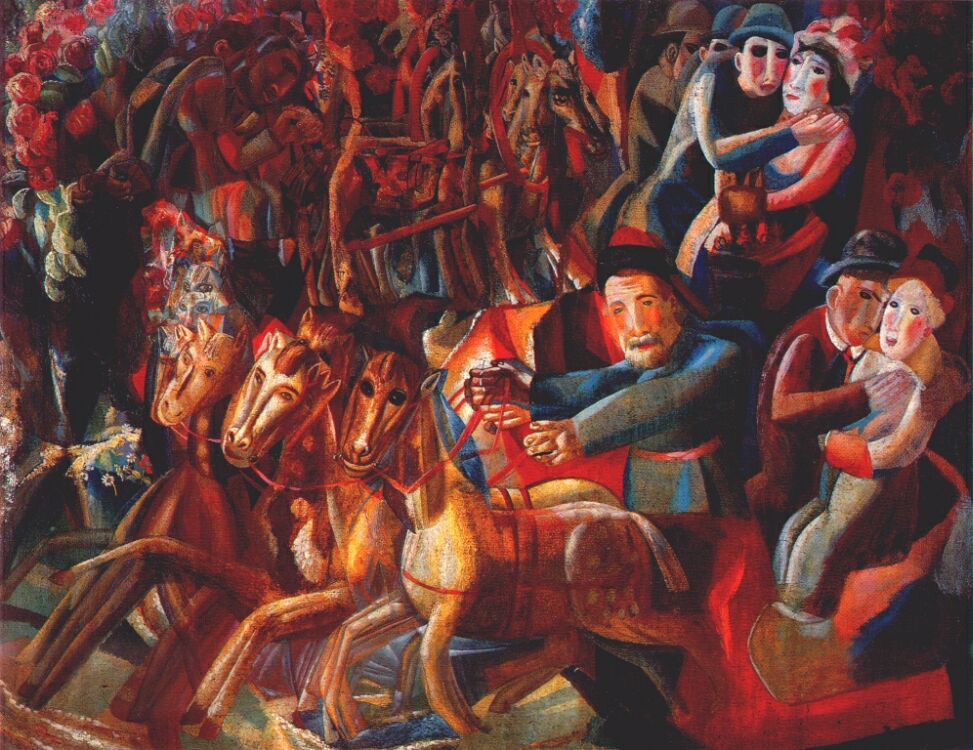The painting is a dramatic and cluttered array of overlapping scenes, predominantly rendered in a color scheme of reds, browns, and blues with dark undertones and orange-yellow highlights. At the upper left, an Indian man with bent elbows and fists near his face appears ready to block a punch. Just below him, three menacing rocking horses with hollowed eyes and tilted heads seem to glare ominously towards the viewer. Behind these eerie horses stands a frightened man in a blue trench coat and red hat, holding the reins and seemingly trying to steer away from them.

In the foreground, lined up hobby horses dominate the scene, directed by a gentleman standing behind them. To the right, two couples are depicted with white faces, red rosy cheeks, and black eye sockets, contributing to the eerie atmosphere. The male figures don hats and are shown embracing their female counterparts, who are repeated in various forms and clothing throughout the painting. The juxtaposition of these unsettling elements creates a visually chaotic and surreal composition, evoking a sense of claustrophobia and tension.